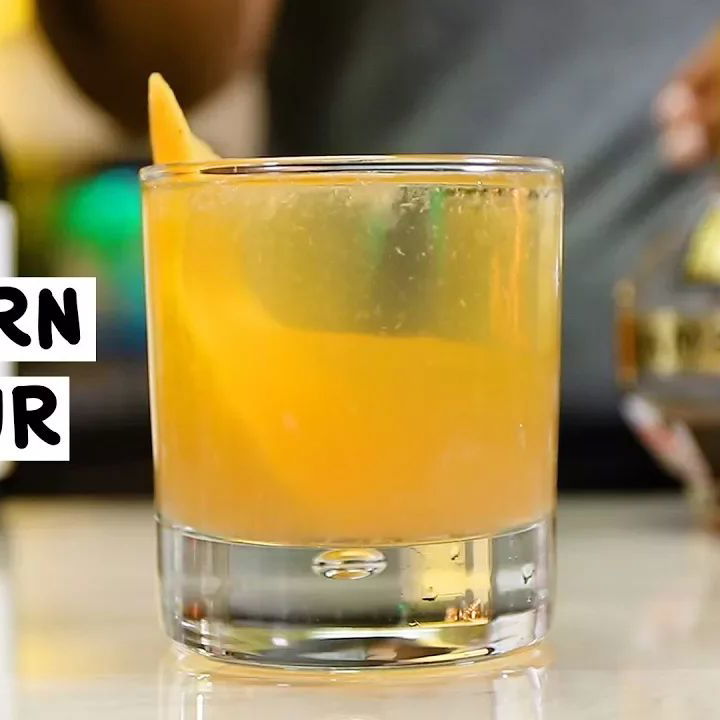The image is a square-format color photograph featuring a cocktail drink prominently positioned on the right side of the frame. The cocktail is contained within a short, clear glass, filled nearly to the brim with an orange-hued liquid, possibly tinged by a garnish of a citrus slice—either lemon or orange—that is partially submerged but extends out over the left edge of the glass. The text "Modern Sour" is elegantly inscribed in black on two horizontal white strips near the center-left of the image. In the more blurred background to the left, there is a larger glass bottle with a dark green tint and a white label, hinting at additional beverage-related elements. Another bright, neon green bottle can be discerned to the right of the dark green bottle, further enriching the context of a beverage-centric setting. The overall style of the photograph is realism, capturing the intricate details and textures of the objects with a representational approach.